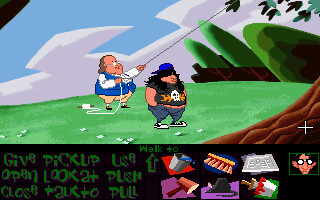In this video game-inspired image, two characters stand prominently in the center. The character on the left, slightly behind and at an angle to the one on the right, bears a striking resemblance to Benjamin Franklin. He is depicted as a short and stout figure with ruddy skin. He is dressed in a blue vest layered over a white long-sleeve shirt, paired with beige knickers and white stockings. His attire is completed with buckled shoes, and his long hair adds to the historical likeness. Notably, he is holding a kite string, with the kite visible in the sky above, adding an element of whimsy and nod to Franklin's famous lightning experiment.